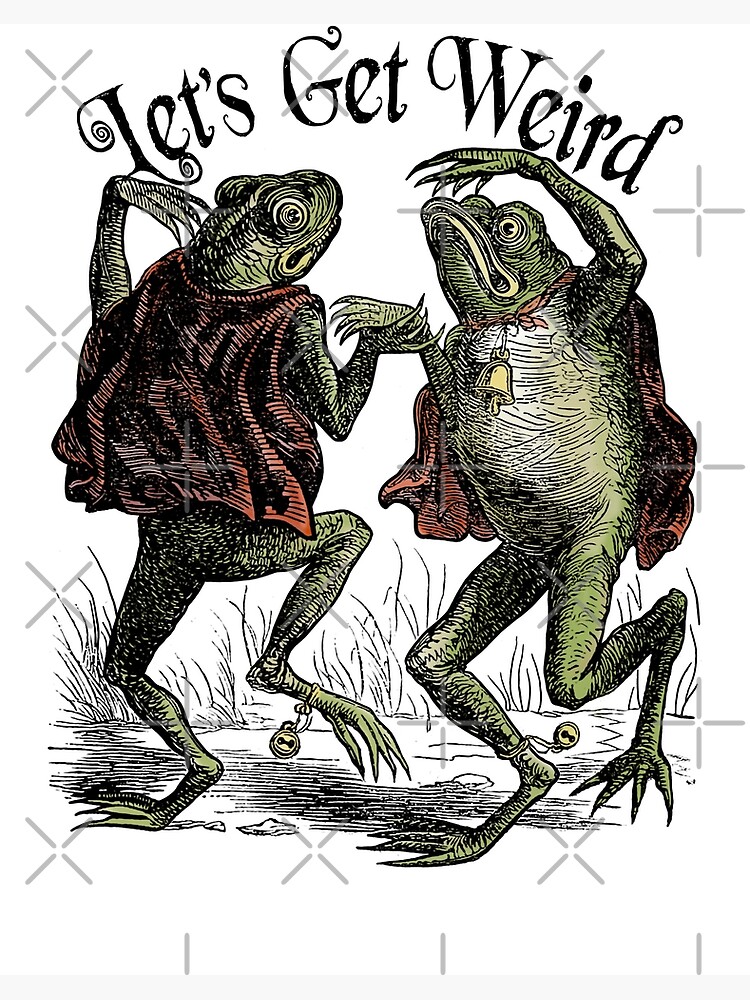In this vibrant illustration, two anthropomorphic frogs are depicted standing upright on their hind legs, holding hands and dancing joyously. They are adorned in red capes that flutter as they move, each cape secured around the neck with a small bell. One frog faces the viewer, clearly displaying its bell, while the other faces away. Both frogs have additional small bells tied to one of their ankles. The frogs are set against a sketched background of sparse grass and shadow, lending a whimsical and somewhat unfinished feel to the scene. Surrounding them are random blue crosses, adding a playful touch. At the top of the image, the phrase "Let's Get Weird" is written in a quirky black font, perfectly encapsulating the eccentric and playful nature of the scene.